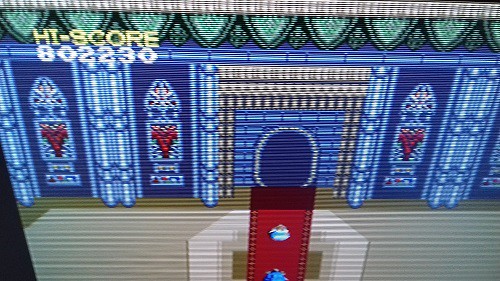A highly pixelated screenshot of an old video game, displaying a grainy, low-resolution image reminiscent of vintage arcade or early home computing screens. The text in the upper left corner, with the words "HIGH SCORE" in a yellowish font, reveals a score of 802230. The background depicts the interior of a room featuring stained glass windows and a central pedestal. The image is characterized by horizontal grainy lines and rough edges, emphasizing its retro aesthetic and the dated technology used to capture it.